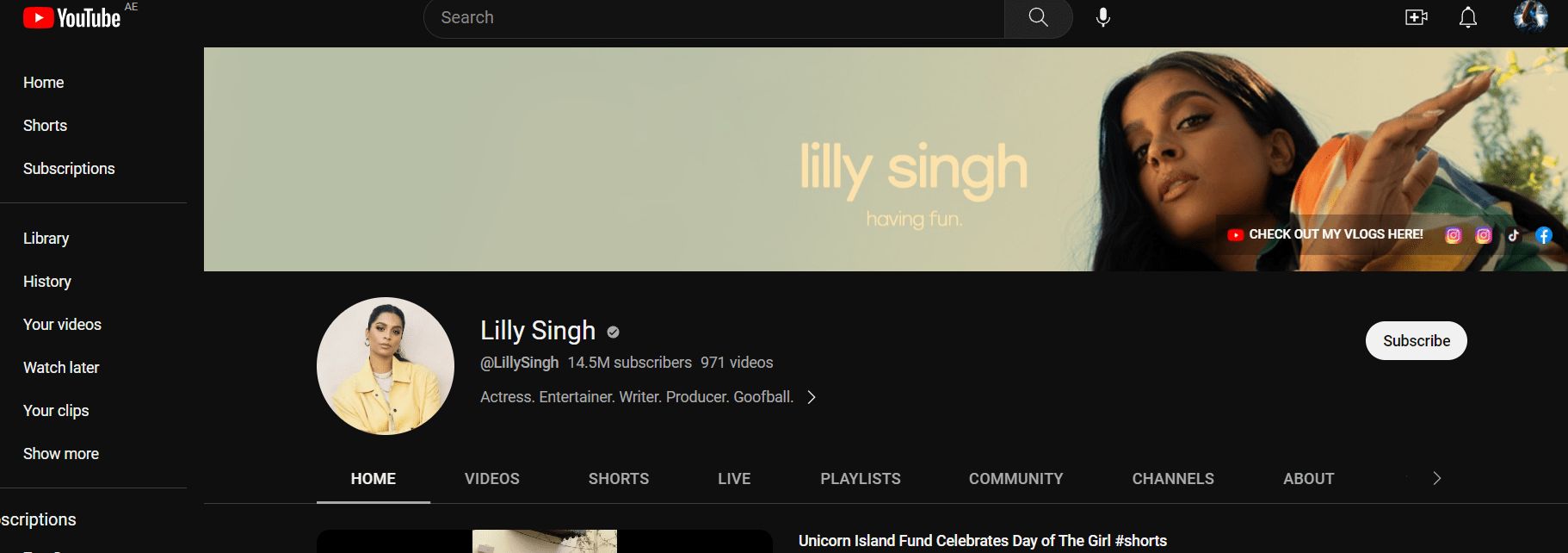Detailed Image Caption:

The image showcases a user interface of the U2 platform on a black background. At the top, there is a long rectangular header. On the left side of the header, the iconic U2 play button is visible, followed by the "U2" text in white. Moving right, a search bar with a magnifying glass icon is centrally positioned next to a microphone icon. Further to the right, there is a battery indicator, a bell notification icon, and an indiscernible icon.

To the very right side, there's a vertical navigation column featuring several options such as "Home," "Shorts," "Subscriptions," "Library," "History," "Your Videos," "Watch Later," "Your Clips," and a "Show More" button.

Adjacent to this column is a prominent light green rectangle featuring an image of Lilly Singh, an Indian woman. Above her picture is the text "Lilly Singh". Below the image, there is a text call-out encouraging viewers to "Check Out My Videos Here," accompanied by links to her Instagram, Facebook, and another unspecified platform. Beneath the image, Lilly Singh's name appears again, followed by symbols, listing "14.5 million subscribers" and "971 videos". Her titles - "Actress, Entertainer, Writer, Producer, and Goofball" - are prominently displayed. To the right of this section is a white "Subscribe" button.

Lower on the page, a series of tabs are visible: "Home," "Videos," "Shorts," "Live," "Playlist," "Community," "Channels," and "About."